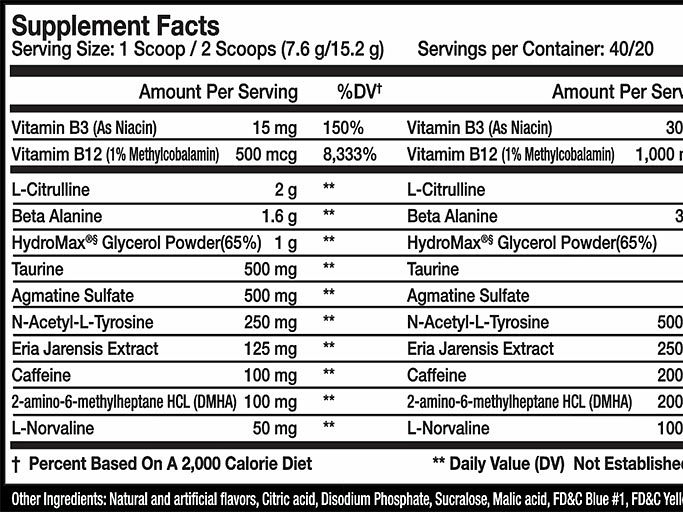This black-and-white nutrition guide appears to be affixed to a dietary supplement, likely a protein or strength-enhancing powder meant to be mixed with water. The label details the supplement facts for both one-scoop and two-scoop servings and indicates that there are 40 servings per container. It lists a range of ingredients and their benefits, including Vitamin B3, Vitamin B12, L-Citrulline, Beta-L-Linolene, HydroMax Glycerol Powder, Taurine, Agmatine Sulfate, N-Acetyl L-Tyrosine, Urea Generis Extract, Caffeine, Aminomethyl Leptin, and Norvaline. Additional notes highlight that the listed percentages are based on a 2,000 calorie diet. The product also contains natural and artificial flavors, citric acid, disodium phosphate, sucralose, malic acid, and FD&C Blue No. 1. This supplement appears to be designed to provide extensive nutritional support, enhancing strength and overall health.